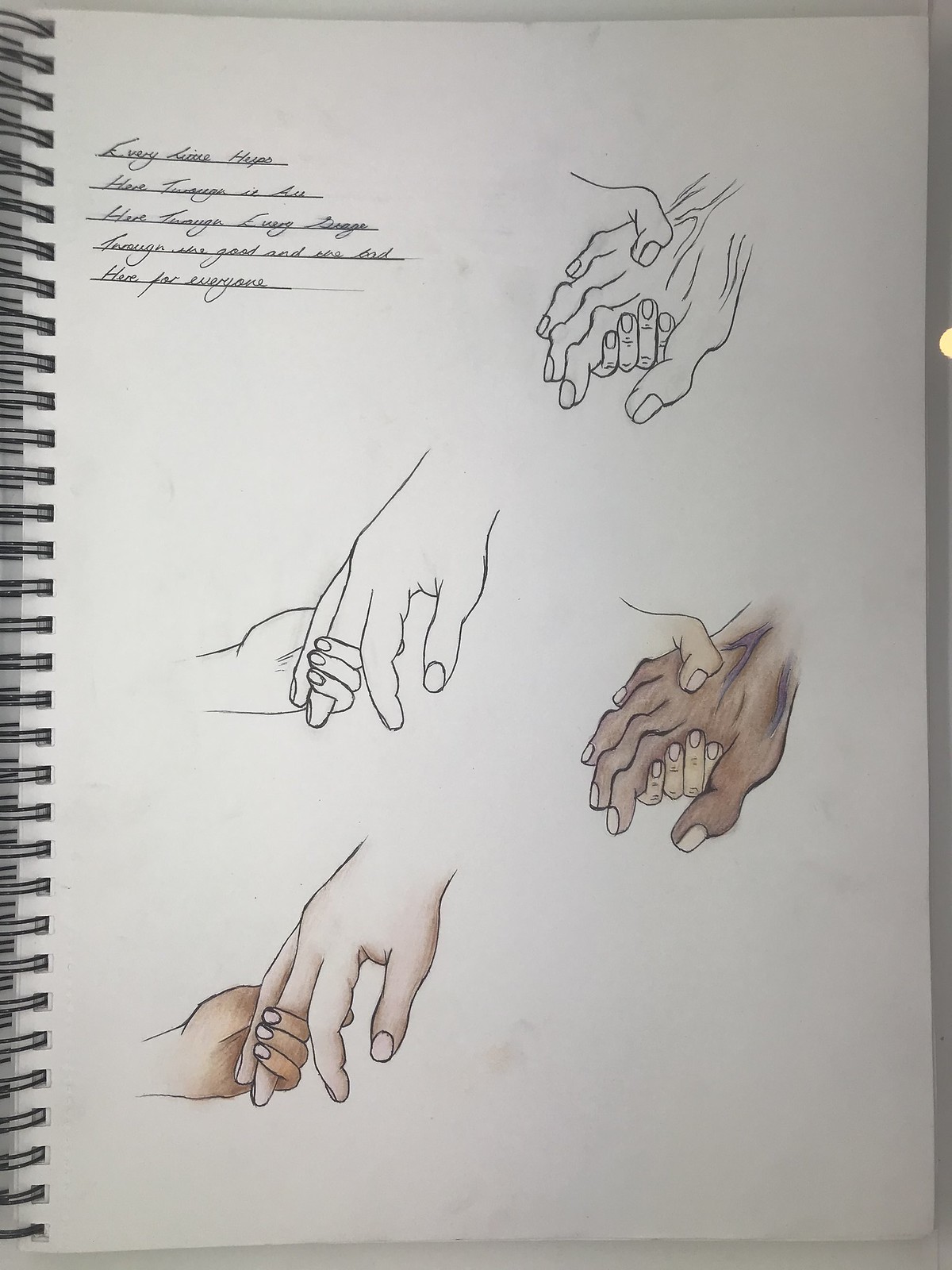This photograph captures a detailed sketchbook illustration, showcasing a series of hand-drawn images. The spiral binding on the left features a continuous loop pattern, giving the notebook a classic and functional appearance. Within the sketchbook, there are four intricate drawings depicting pairs of hands. 

In two instances, an older, wrinkled hand is tenderly clasped by a younger, smoother hand, symbolizing care and generational connection. The other two sketches illustrate an adult hand being held by a child's much smaller hand, emphasizing protection and nurturing. The child’s hand is delicately gripping a couple of the adult's fingers, portraying tenderness and dependency.

Above these evocative drawings, a message is written in small, slanted, and tightly packed text. Though challenging to decipher, it reads: "Every line helps here through every day, here for everyone." Each line of the text is underlined, presumably to emphasize its importance, though the crowded nature of the writing slightly obscures the clarity. This thoughtful composition combines meticulous artistic detail with a poignant narrative.